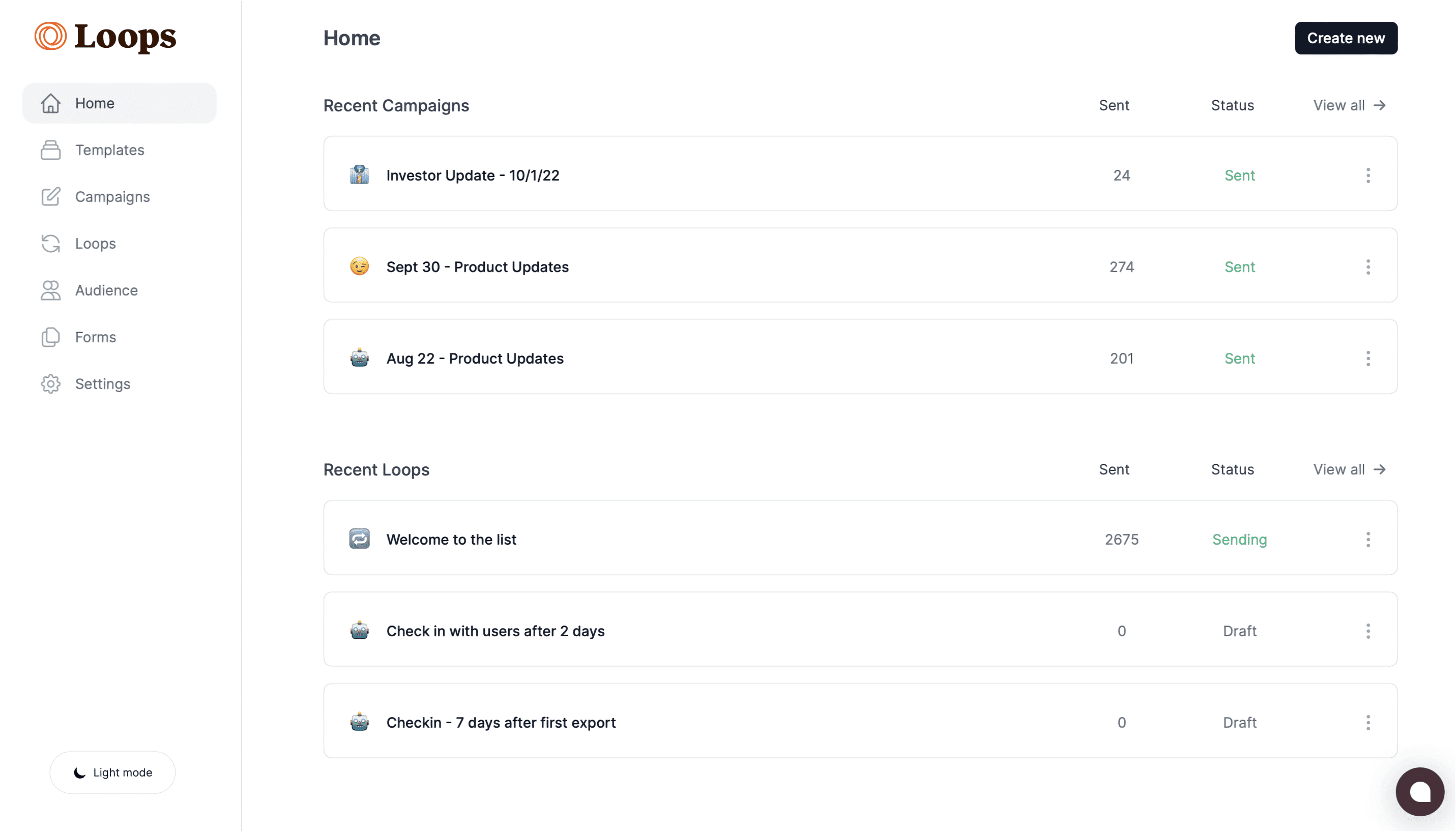The clean and detailed caption for the image would be:

"The website features a minimalist white background. In the top left corner, there is a distinctive logo composed of interlocking red circles that create a pattern reminiscent of tire tread or a spiral. The center of the logo is white. To the right of the logo, the word 'Loops' is prominently displayed in bold black letters. 

Below the logo is a vertical menu with several clickable options. The first option, highlighted in light gray, includes a little home icon and the word 'Home.' Following this are other icons and labels in black text: 'Templates' with a template icon, 'Campaigns' with a square and pencil icon, 'Loops' with a circle and two arrows icon, 'Audience' with two profile icons, 'Forms' with overlapped squares icon, and 'Settings' with a gear icon. 

In the bottom left corner of the menu, there is a quarter moon icon labeled 'Light Mode.' Just to the right of 'Loops,' the word 'Home' appears again. On the right side of the page, there is a black tab with 'Create New' written in white lettering. 

Below 'Home,' a section labeled 'Recent Campaign' is displayed. To the right of this, an arrow pointing to the right with the text 'View All' is visible, with 'Status' and 'Sent' labels beneath it. 

Under the 'Recent Campaign' section, there are three small icons followed by three clickable tabs. The 'Sent' numbers and their statuses are indicated, telling whether they are sent or drafted. Another section labeled 'Recent Loops' appears below, featuring three more icons with similar status indicators and a 'View All' option to the right.

Finally, in the bottom left corner, a black circle containing a small white circle adds to the minimalistic interface design."